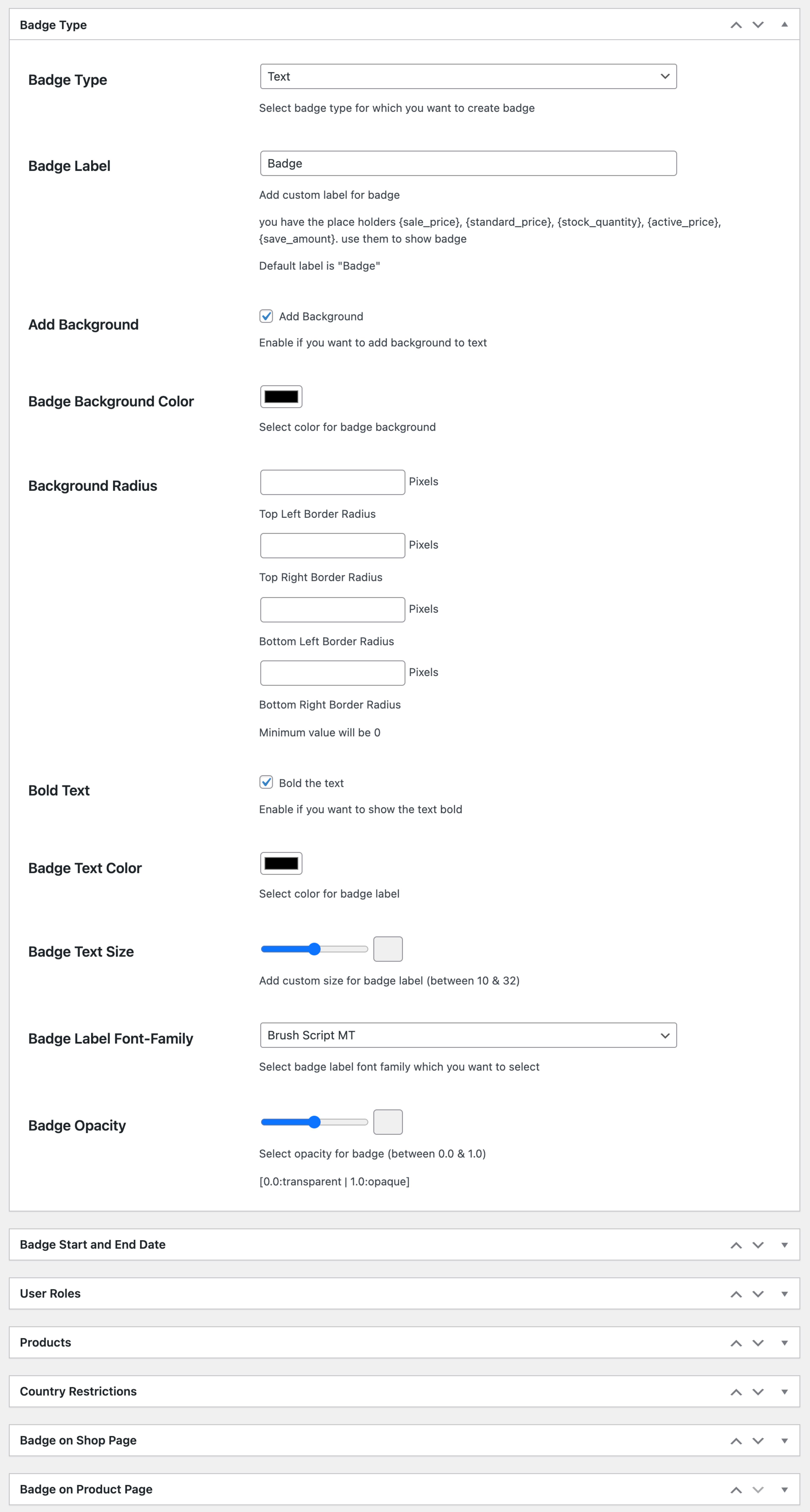The image is a detailed screenshot of a user interface for configuring badge types within a software program. The interface has a clean, white background, and at the top-left corner in small black letters, it reads "Badge Types." The top-right corner features icons for an upward arrow, a downward arrow, and an "X" for closing the window.

On the left side of the page, various categories are listed. On the right side, for each category, there are option titles, input boxes, dropdown menus, and other actionable elements. 

The detailed customization options include:

- **Badge Type:** A dropdown menu with "Test" selected.
- **Badge Label:** A text box with the word "Badge" entered.
- **Add Background:** A checkbox to enable or disable adding a background. This checkbox is selected.
- **Badge Background Color:** A small clickable box for color selection, with black currently selected.
- **Background Radius:** Four separate input boxes to define the dimensions of the background's corners.
- **Bold Text:** A checkbox to toggle bold text; this box is checked.
- **Badge Text Color:** A color selection box currently set to black.
- **Badge Text Size:** A slider positioned halfway across its range.

Additional customization options are listed further down the page.